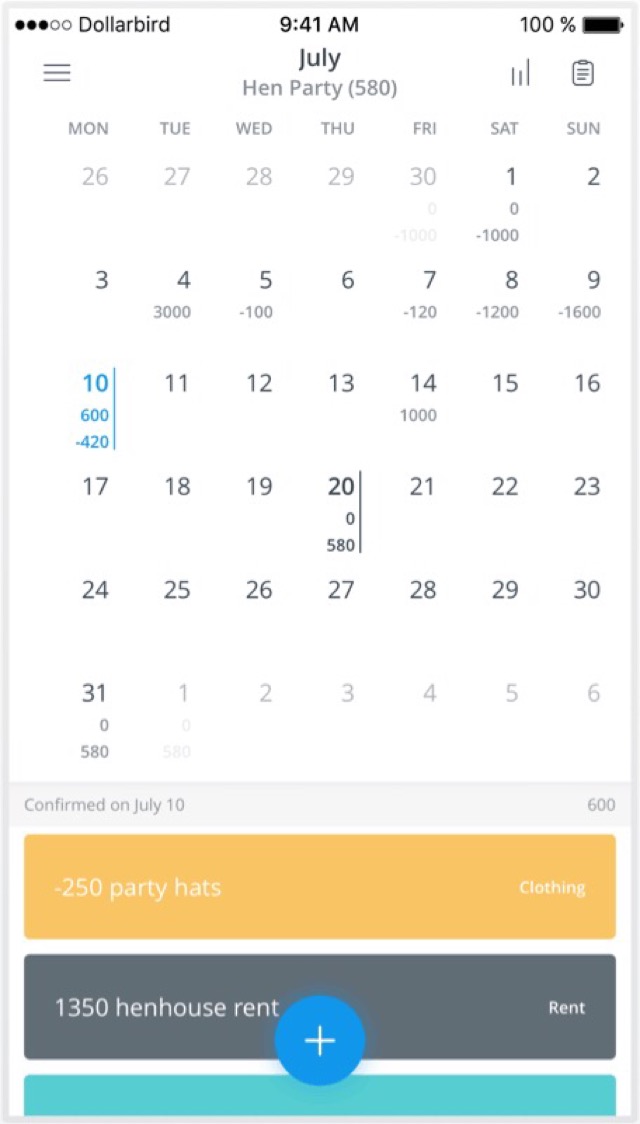This photo captures the calendar app on a smartphone, displaying the month of July. On the left side of the screen, there are three out of five filled circles, and the word "Dashboard" is prominently displayed at the top center of the screen. The current time is shown as 9:41 a.m., and the battery indicator on the far right shows a full charge at 100%.

The calendar view starts with the last few days of June, specifically the 26th to the 30th, flowing into the entirety of July, numbered from 1 to 31. Under the heading "July," an event titled "Hen Party 580" is visible. At the screen's bottom, a tan bar indicates "250 party hats and clothing," while a dark blue bar beneath it denotes "1350 in-house rent." Centered at the bottom is a blue circle with a plus sign, presumably for adding new entries. Partially visible below this is another bar, which is cut off in the image, providing an additional hint of the app's interface and functionalities.